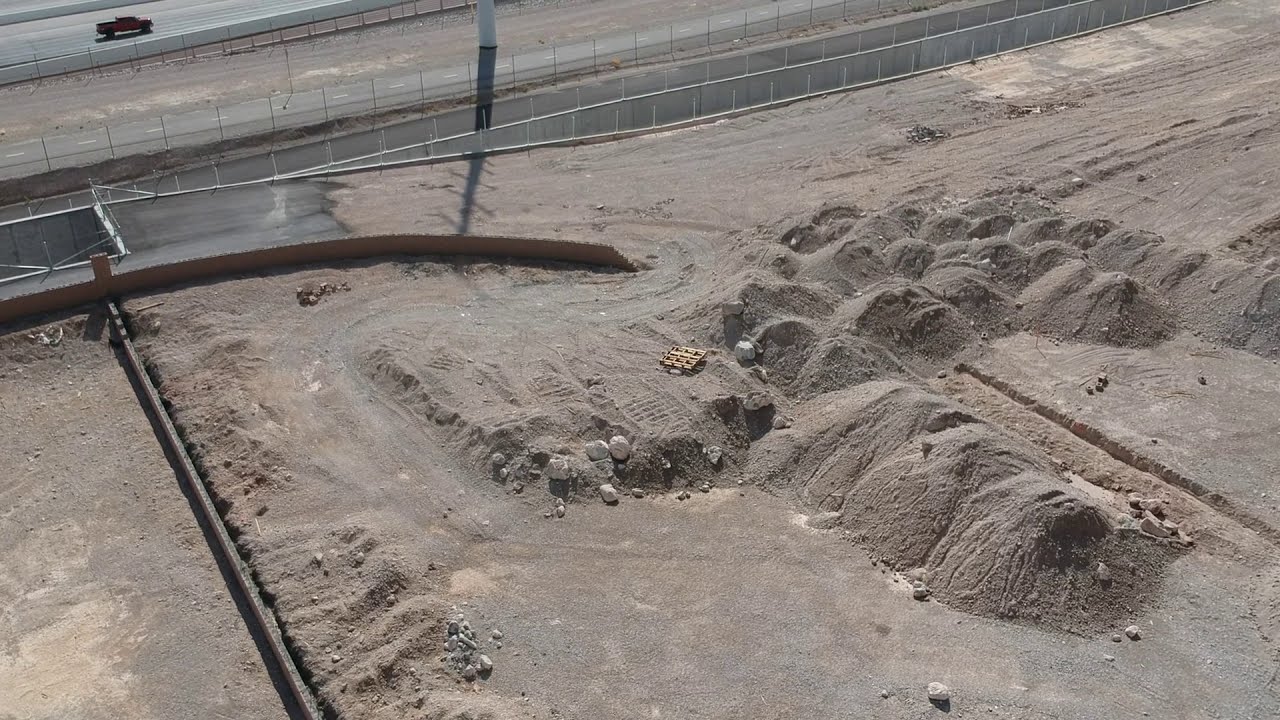This aerial digital photograph, taken during the daytime, showcases a bustling construction site where the foliage has been entirely cleared. The focal point of the scene is a gravel and sand work area featuring multiple substantial piles of sand and dirt. On the right-hand side, the terrain is uneven with numerous bumps and dips, while the left-hand lower corner reveals a freshly dug trench with a laid foundation and a flattened area adjacent to it. Surrounding portions of the site, large boulders are strategically placed. 

The upper left-hand corner of the image captures a truck journeying from left to right on a two-laned highway, visually segregated from the construction zone by a fence line. The site is partitioned by multiple fences, providing barriers between the roadways and the work site. The vivid colors of brown, red, white, and gray dominate the landscape, emphasizing the site's industrial nature.